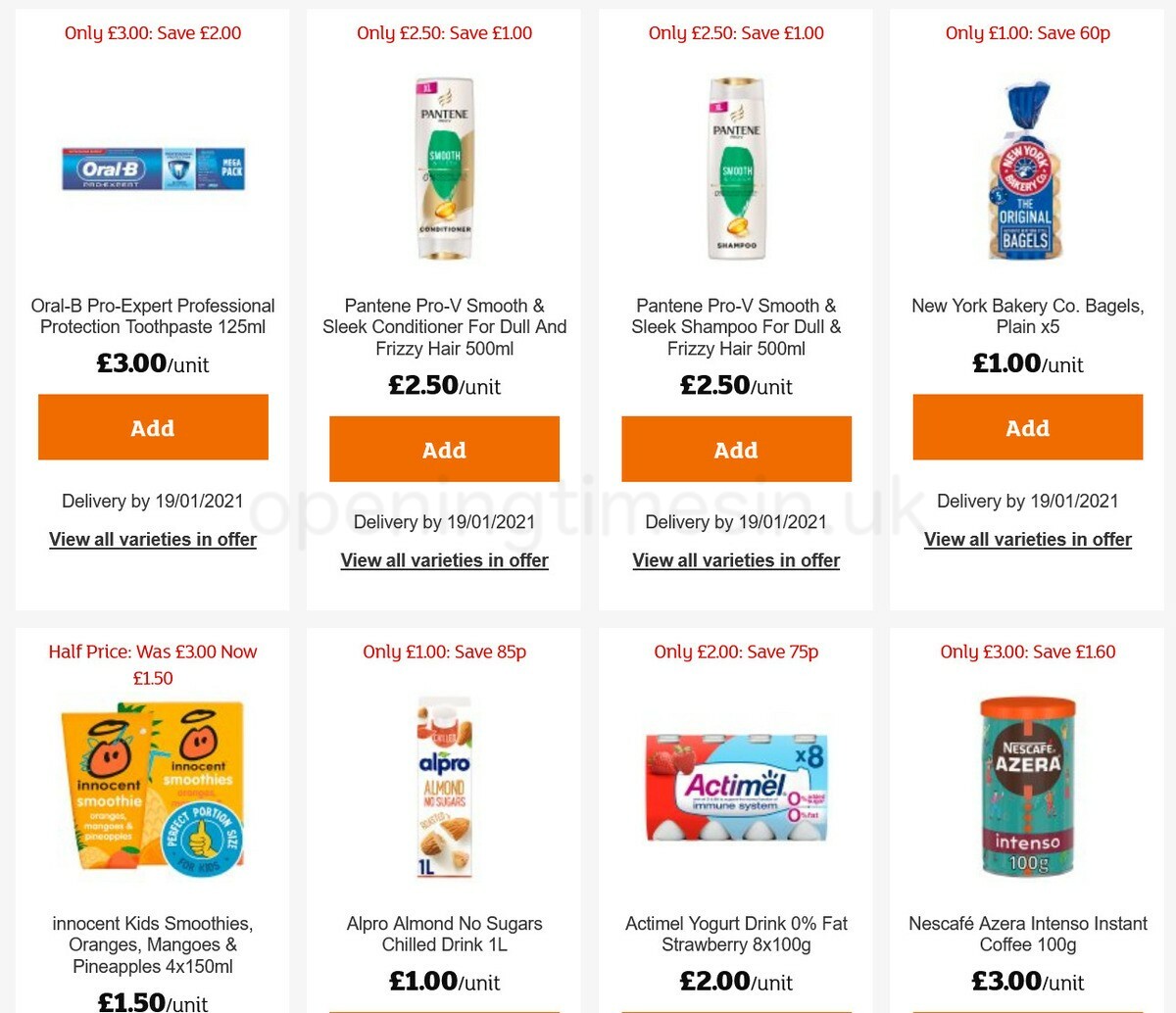This image is a detailed screenshot of a promotional advertisement featuring various products with discounted prices. 

### Top Row:
1. **Oral-B Pro-Expert Professional Protection Toothpaste**
   - **Price**: Only £3, save £2
   - **Details**: Each unit is priced at £3. An "Add to Cart" option is available.
   - **Visual**: An image of the Oral-B toothpaste.

2. **Pantene Pro-V Smooth and Sleek Conditioner**
   - **Price**: £2.50, save £1
   - **Details**: Specifically for dull and frizzy hair. An "Add to Cart" option is available.
   - **Visual**: An image of the Pantene conditioner bottle.

3. **Pantene Pro-V Smooth and Sleek Shampoo**
   - **Price**: £2.50, save £1
   - **Details**: Specifically for dull and frizzy hair. An "Add to Cart" option is available.
   - **Visual**: An image of the Pantene shampoo bottle.

4. **New York Bakery Co Bagels**
   - **Price**: Only £1, save 60p
   - **Details**: An "Add to Cart" option is available.
   - **Visual**: An image showing a bag of bagels.

### Second Row:
1. **Tea Bags**
   - **Price**: Half price, was £3, now £1.50
   - **Details**: An "Add to Cart" option is available.
   - **Visual**: No specific brand or image description provided.

2. **Innocent Kids Smoothies**
   - **Price**: Now only £1, save 85p
   - **Details**: Flavors include oranges, mangoes, and pineapples. An "Add to Cart" option is available.
   - **Visual**: No specific image description provided.

3. **Alpro Almond No Sugars Drink**
   - **Price**: Only £2, save 75p
   - **Details**: A plant-based drink. An "Add to Cart" option is available.
   - **Visual**: Not explicitly described.

4. **Actimel Yogurt Drink 0% Fat Strawberry**
   - **Price**: Only £3, save £1.60
   - **Details**: An "Add to Cart" option is available.
   - **Visual**: An image showing a pack of Actimel yogurt drinks.

5. **Nescafe Azera Intenso Instant Coffee**
   - **Price**: Only £3, save £1.60
   - **Details**: An "Add to Cart" option is available.
   - **Visual**: An image of a can of Nescafe Azera Intenso instant coffee.